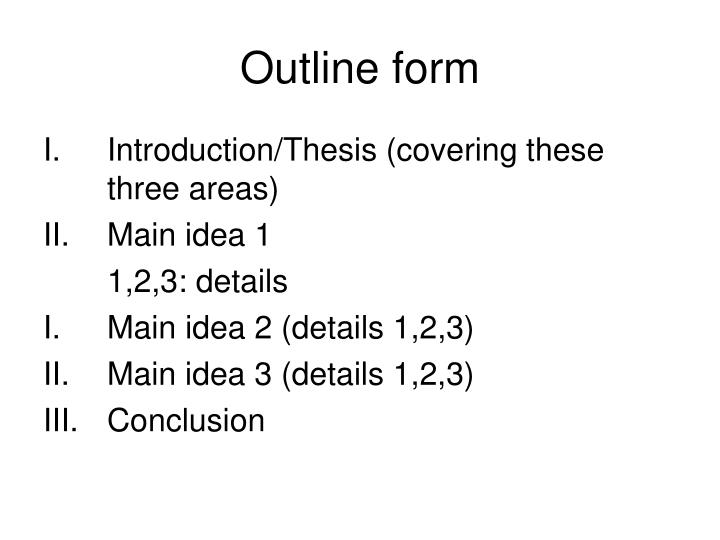The descriptive caption for the image would be: 

This black and white outline form is presented on a plain white background with no discernible border. The centered header with the larger font reads "Outline Form." Below the header, the text is aligned on the left and structured with Roman numerals. The outline starts with "I. Introduction / Thesis (covering these three areas)," followed by "II. Main Idea 1," and beneath it, indented, "1, 2, 3 - details." Continuing, "III. Main Idea 2 (details: 1, 2, 3)," and next is "IV. Main Idea 3 (details: 1, 2, 3)." The final point is "V. Conclusion." The entire layout resembles a structured format, likely intended for a PowerPoint presentation, with the title positioned at the top and the text below, centered and slightly off to the left. The presentation of the text in black font against a white background emphasizes clarity and simplicity in the outline's format.